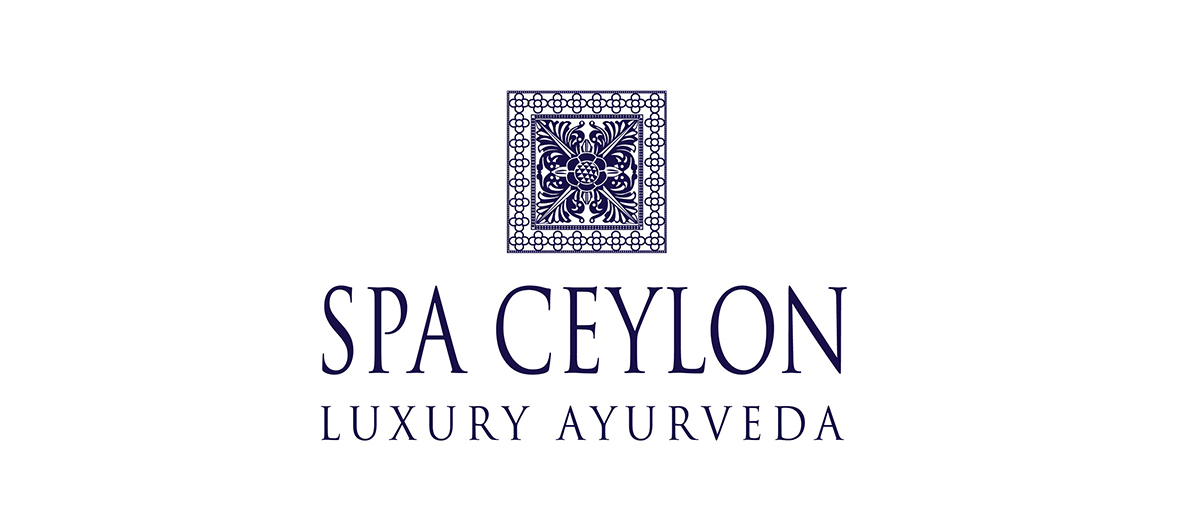This advertisement features a visually striking logo for "SPA CEYLON" in bold, large uppercase black font at the bottom of the frame, with "Luxury Ayurveda" written beneath it in smaller uppercase font. Above the text is a square logo with intricate details: it consists of an outer square surrounding a smaller inner square, separated by a border adorned with a repetitive shamrock or Celtic cross pattern. Within the inner square, there is a black and white drawing featuring a symmetrical X pattern created by a pair of diagonal elements, potentially resembling swords or plant stems, and a circular design at the center. The entire image stands against a clean, plain white background, emphasizing the elegance and intricate details of the SPA CEYLON Luxury Ayurveda branding.